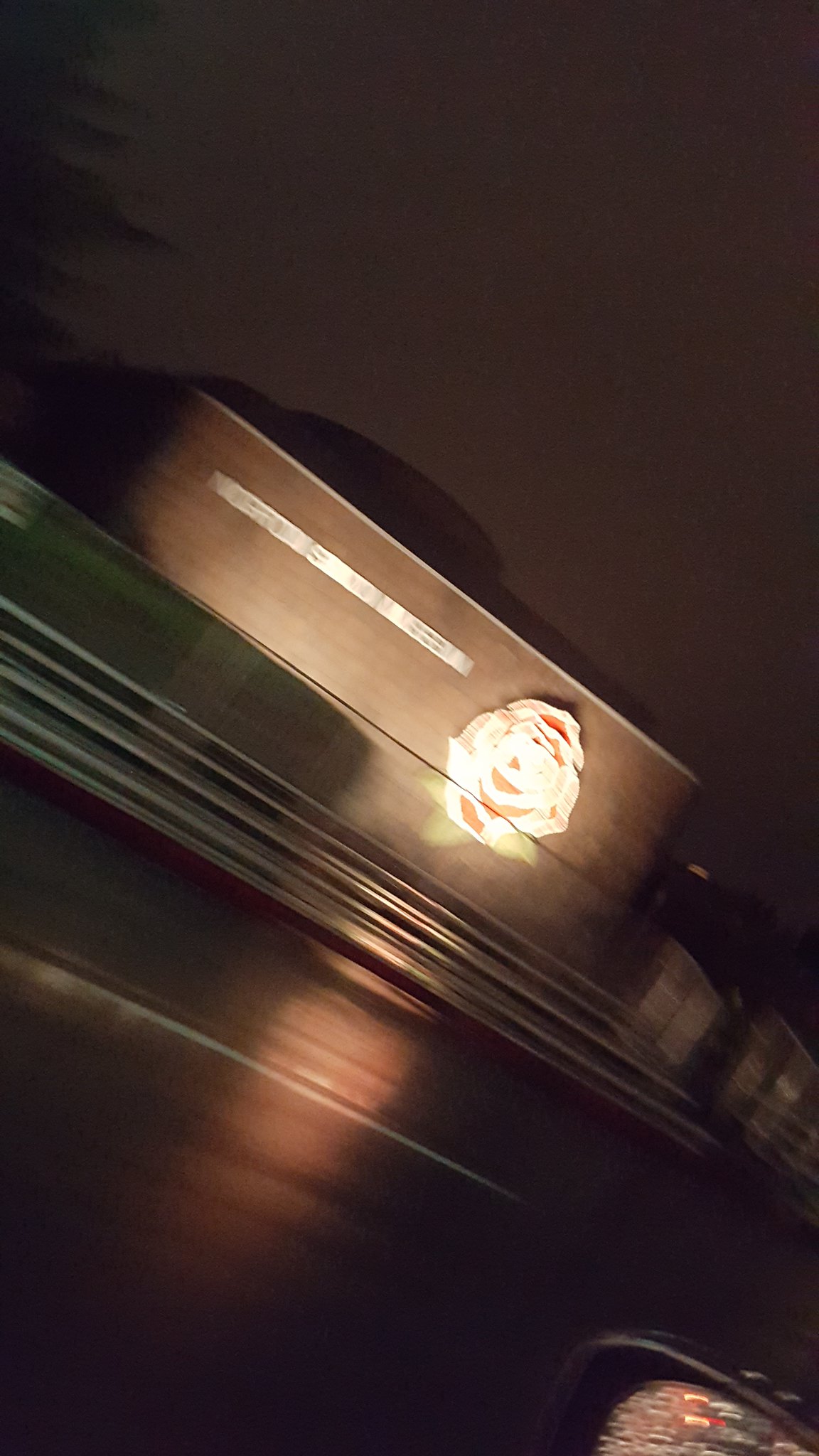This nighttime, slightly blurred photo features a tilted composition with a predominantly dark background. Dominating the foreground, which occupies the lower left corner and the bottom of the frame, is a brown wooden surface. Above this, extending toward the upper right corner but still near the center, is a medium brown rectangular object with rounded corners. The object, which appears to be a box, displays one row of white text across it, though the text is indistinct due to the blur.

Distinctly visible on the box is a large ornamental rose motif, which seems embossed as it appears slightly raised from the surface. The rose is mostly white with accents of gold, including three gold leaves, and areas of red. Despite the blur, the rose motif remains clearly identifiable. The image provides no other significant details beyond this decorative box against the dark backdrop.